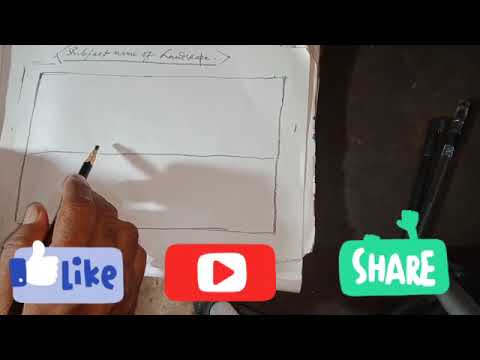This image appears to be a screenshot of a YouTube video depicting a close-up view of a right hand, notably tanned or light-mixed race, holding a black pen or pencil over a white sheet of paper. The hand is poised to draw on the paper, which features two rectangular boxes, one above the other. The top of the paper has some unclear, blurry text that might refer to "subject matter of landscape." The setting suggests the person is indoors, under lighting that casts shadows onto the paper. To the right of the paper, a black pen with its cap on is visible against the dark black wood of the desk. The image has black bands at the top and bottom, contributing to a somewhat grainy, older video quality. Superimposed at the bottom are three cartoonish buttons: on the left, a blue "Like" button with a thumbs-up icon; in the middle, a red YouTube-like button with a play icon; and on the right, a green "Share" button with white text, alongside a hand icon. The overall color scheme includes brown, black, white, light purple, red, and light green.